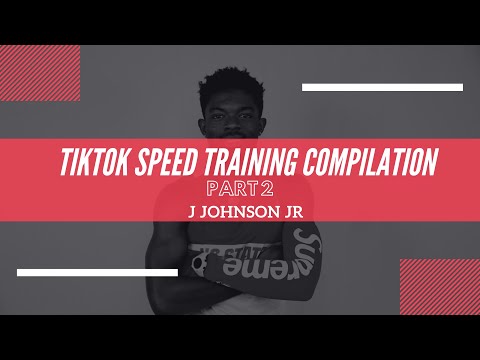The image features a monochromatic gray background with a text overlay in a red box situated at the upper left and lower right corners. These corners also contain decorative horizontal lines. At the center of the image stands a young man, presumed to be an athlete, wearing a unique jersey with text on the chest and left sleeve. His arms are crossed and he poses confidently. Prominently displayed in the red box is the white text: "Tick Tock Speed Training Compilation Part 2, Jay Johnson Jr." The image appears to be a promotional screenshot from a TikTok video, where the overlaid text likely fades away to reveal more of the young man's actions or discourse.